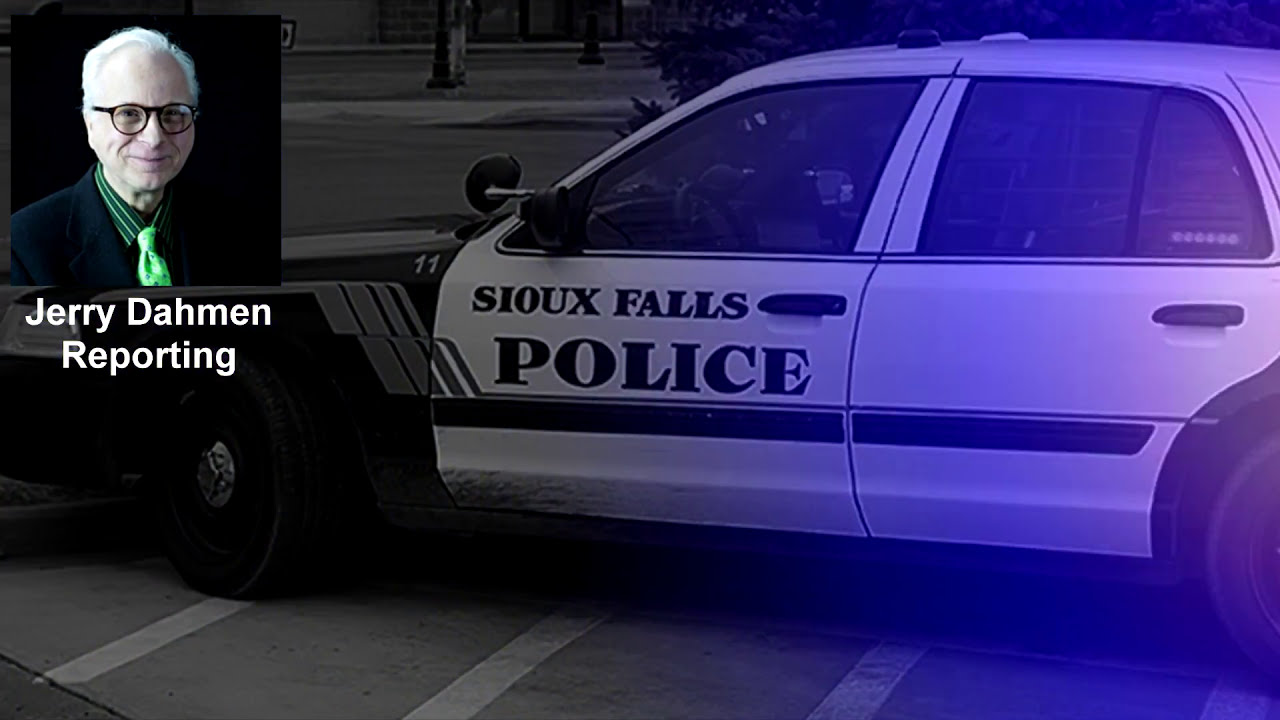The image features a Sioux Falls Police car with a distinctive black and white color scheme, having white doors and roof, and a black front fender and hood. The car, marked with the number 11 in the upper corner of the fender, displays bold black text on its white door that reads "Sioux Falls Police," alongside a black strip running horizontally underneath. The half-parking, half-driving vehicle is captured in a landscape layout, cutting off at the back wheel, with the front facing left and the back extending towards the right. The background of the image transitions from a dark hue on the left to a blue hue on the right.

In the upper left corner of the image is a photograph of an older white man with white hair. He wears black glasses with round rims, a black shirt, and tie. This man, identified by white text below the image as "Jerry Dahman reporting," appears with smiling facial expressions in some descriptions and without facial hair. The altered consistency in his attire across the descriptions includes references to a green tie and a black jacket. Beneath the police car are four painted white stripes stretching diagonally from the upper right to the lower left, suggesting a parking lot from where the car seems to be pulling out onto the street.